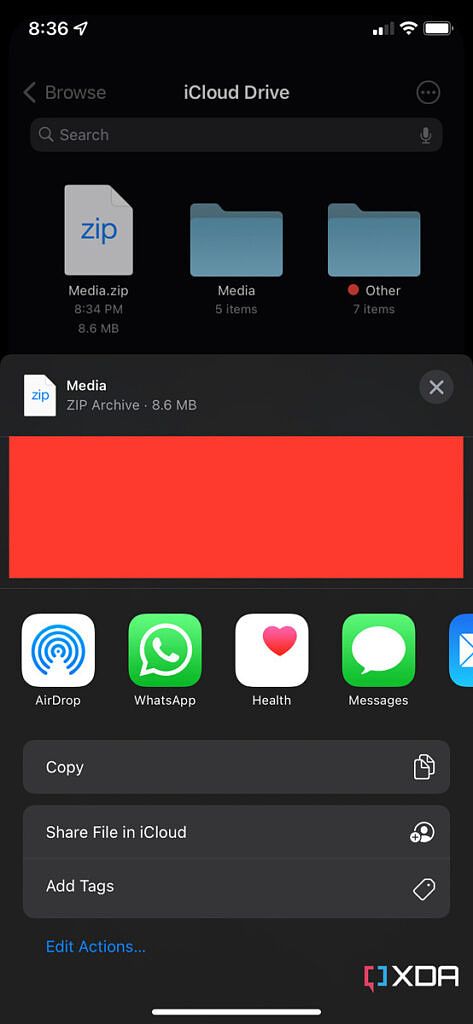In the image, a user is navigating their Apple iPhone interface, clearly identifiable by the presence of the iCloud feature. The screen background is black with white text, providing a clean contrast. 

At the top left corner, the time is displayed as 8:36 a.m., while the top right corner shows the device's battery at 50% with a strong Wi-Fi connection icon. 

Centered below these indicators is the title "iCloud Drive," highlighting that the user is managing their cloud storage. To the left of this title is a slightly faded "Browse" button accompanied by a left arrow, indicating a navigation option.

Directly beneath the title bar is a search field with a magnifying glass icon and a microphone icon, suggesting the option to type or voice input search queries.

The main content area lists three different files:
1. A white document icon labeled "media.zip" saved at 8:34 p.m., with a file size of 8.6 MB.
2. A blue folder labeled "5 items," indicating it contains multiple files.
3. Another blue folder labeled "7 items."

Below these items, there's an interface element allowing the user to exit the screen. 

Further down, a line of application options appears, including "Airdrop," "WhatsApp," "Health," and "Messages," each represented by their respective icons. Additional options such as "Copy," "Share File on iCloud," "Add Tags," and "Edit Actions" are aligned towards the bottom left in blue text. Finally, the bottom right corner features an "XDA" logo, denoting a possible source or associated application.